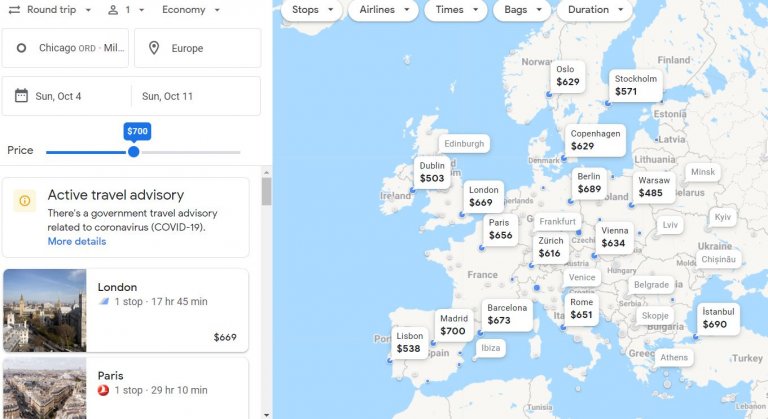**Caption:**

The top left corner of the image displays information for booking a roundtrip economy flight from Chicago, scheduled for Sunday, October 4th, with a return on Sunday, October 11th, priced at $700. An active travel advisory related to COVID-19 issued by the government is also indicated in the image. 

The destinations and flight details include:

- **London:** 1 stop, 10 hours 45 minutes, $669.
- **Paris:** 1 stop, 10 hours and 20 minutes, $656.
- **Oslo:** Direct, priced at $629.
- **Stockholm:** Direct, priced at $571.
- **Copenhagen:** Direct, priced at $629.
- **Dublin:** Direct, priced at $503.
- **Zurich:** Direct, priced at $669.
- **Warsaw:** Direct, priced at $645.
- **Vienna:** Direct, priced at $664.
- **Istanbul:** Direct, priced at $690.
- **Rome:** Direct, priced at $651.
- **Barcelona:** Direct, priced at $672.
- **Madrid:** Direct, priced at $700.
- **Lisbon:** Direct, priced at $438.

The background color of the image is blue, highlighting various destinations and flight options across Europe, including countries like Norway, Finland, Estonia, Latvia, Belarus, Turkey, and Greece.